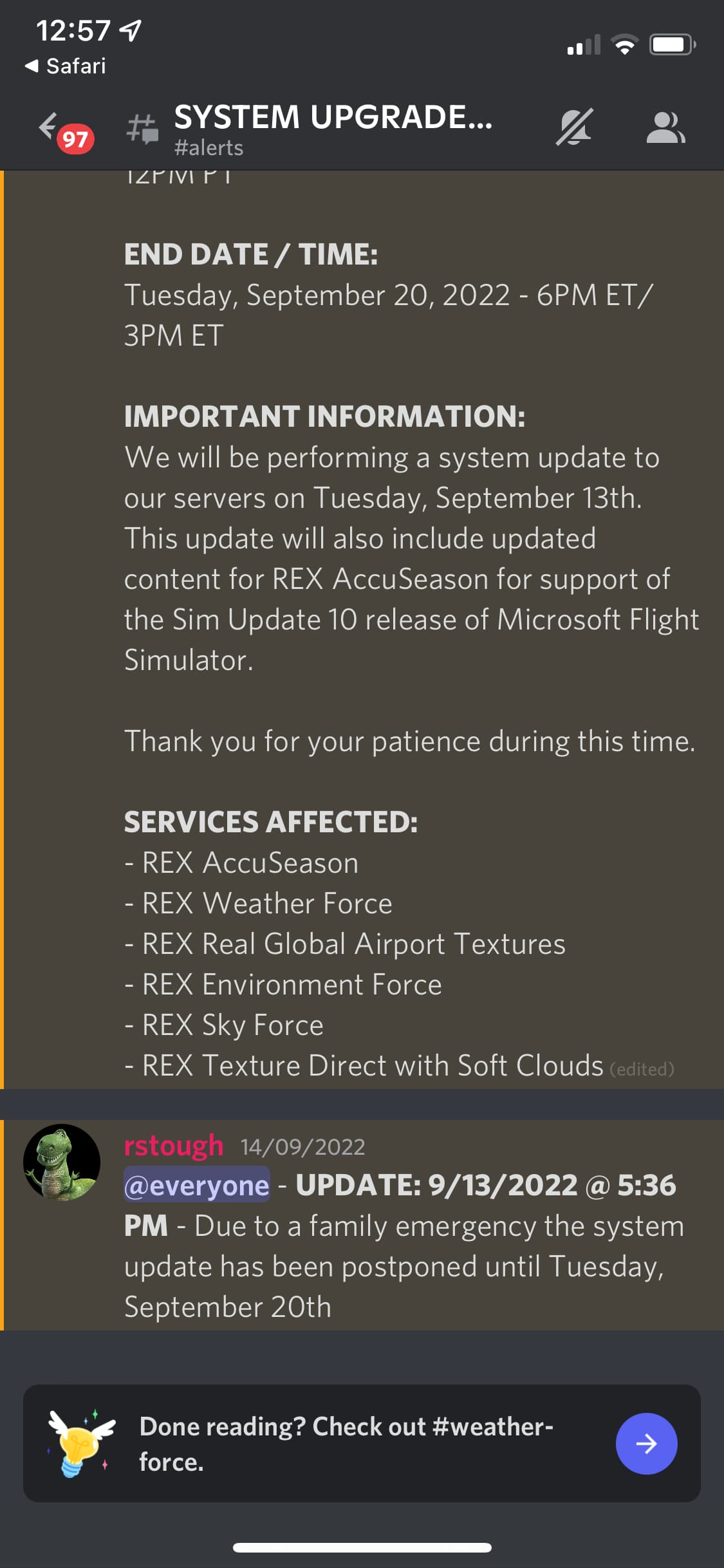**Caption:**
A screenshot capturing a detailed system upgrade alert on an iPhone. The status bar at the top shows the time as 12:57, with 2 out of 4 bars of cellular signal, 2 out of 3 WiFi bars, and a battery at approximately 90%. The device is using the Safari browser, indicated by the browser frame visible in the screenshot. Notifications are muted, denoted by the bell icon with a strike-through, and there are 97 unread messages shown by the person's icon.

The main content is a system update notification scheduled for Tuesday, September 20th, 2022, from 6 PM to 3 PM Eastern Time. It details an upcoming server update with additional content for "rex accu season" in support of the Microsoft Flight Simulator Sim Update 10. A partial scroll reveals gray fields and date and time specifications, emphasizing the importance and duration of the maintenance.

A message panel within the screenshot, which appears to be from Discord, shows an update from the handle @everyone, noting that due to a family emergency, the system update initially scheduled for September 13th has been postponed to September 20th. The message concludes with a call to check the #weather-force channel, indicating the update pertains to weather management tools for the flight simulator.

Services affected include:
- rex accuSeason
- rex Weather Force
- rex Real Global Airport Textures
- rex Environment Force
- rex Sky Force
- rex Texture Direct with Soft Clouds